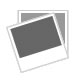The photograph depicts a partially visible, intricately carved wooden door or panel set in the scratched, black plastic bed of a pickup truck. The wooden piece, likely an element of aged furniture, features detailed floral and leaf engravings. Positioned towards the right, the subject showcases a rich, varnished brown hue with layered paint. A border along the left edge is adorned with an ornate leaf and flower design. Toward the center, there is a recessed area with a scroll motif and a small hole located at the top left. The image is cropped, showing only part of the truck bed and a fraction of the wooden piece, leaving much to the imagination about the item's full form and function.